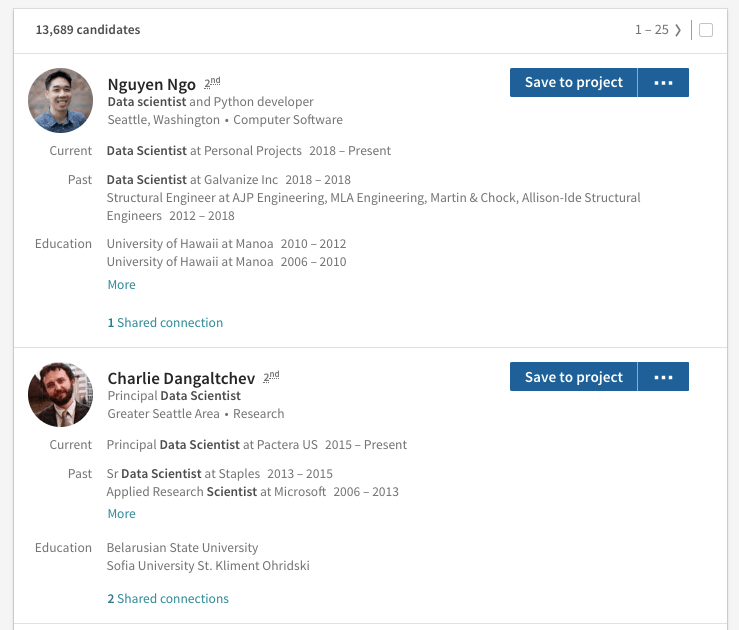This image is a screenshot of a webpage displaying information about two candidates. At the top left, there is a text indicating "13,608 non-candidates." On the right side, navigation options display "1 through 25," along with a forward button. Adjacent to these options is a checkbox.

The first candidate's profile is displayed prominently below these elements. Their profile picture is visible alongside detailed information. At the top left of the profile section, it is noted as "Name: New Dream, No, Second." In the top right corner, there is a blue button labeled "Save to Project," and next to it is a "More info" button represented by three vertical dots.

The profile also contains additional details including their current location, "Seattle, Washington," and their field, "Computer Software." Furthermore, sections for "Current and Past Jobs," and "Education" are listed with an option button to view more information. At the bottom of the profile, it mentions "One Shared Connection."